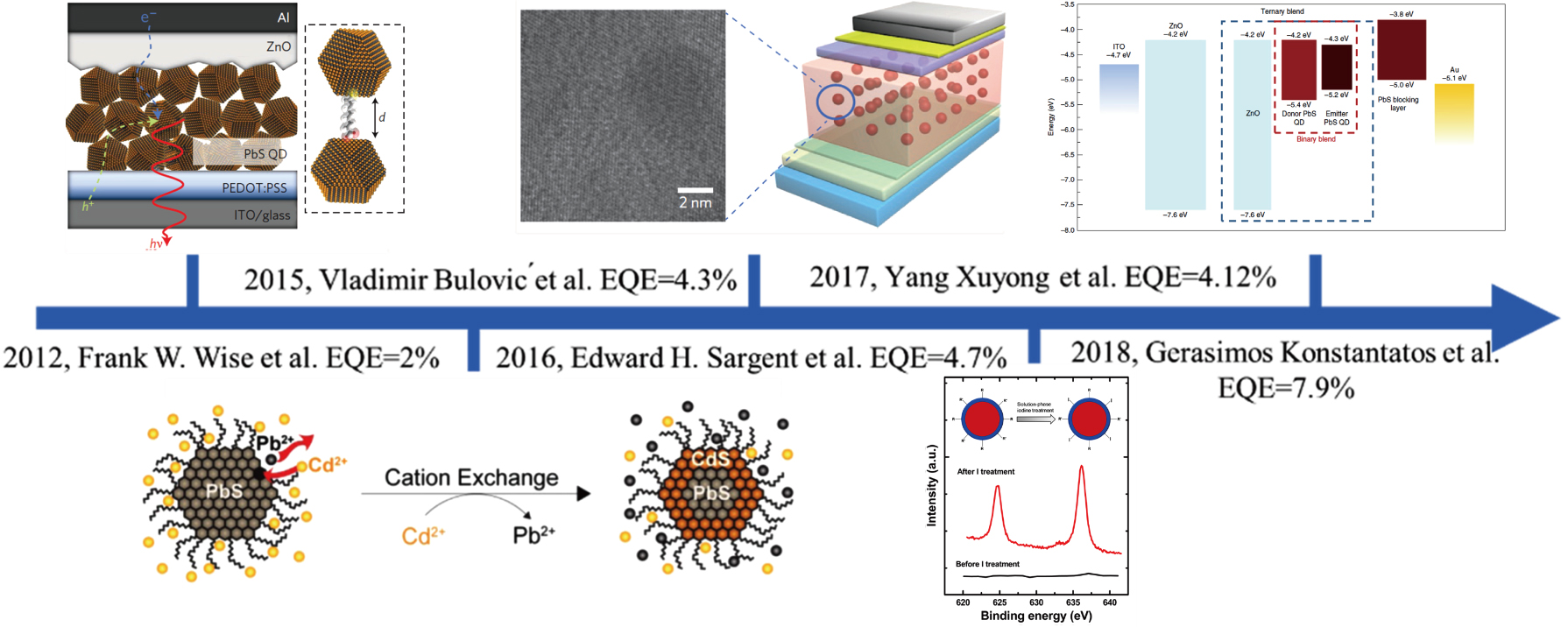This landscape-oriented illustration appears to be a scientific timeline marked by a prominent blue arrow running horizontally from left to right through the center. Key milestones are showcased with detailed images and data:

- At the top left, under "2015 Vladimir Bolivic et al. EQE = 4.3%," there are octagon shapes in brown with black stripes. Near this, a blue vertical line extends up and down from the arrow. A gray square with white '2 MM' lies next to another blue line, linked by dotted lines to a pink box with multiple tiny items, symbolizing layers of these items.
  
- Beneath the arrow, marked "2012 Frank W. Wise et al. EQE = 2%," is a six-sided figure suggestive of a chemical structure, labeled 'Pb,' with small arms extending out. To its right, another blue line points to "2016 Edward H. Sargent et al. EQE = 4.7%" and another similar hexagonal chemical illustration.

- Further right, a square poster featuring two red circles is connected to a blue line above. Below these circles is a line graph labeled "2018 Gerasimos Constantatos et al. EQE = 7.9%."

- Following the top-right segment, "2017 Yang Zhuang et al. EQE = 4.12%" includes a gray square connected to a pink box via dotted lines, symbolizing the association of different layers.

- Adjacent is another visual incorporating bar graphs—light blue, red, burgundy, and yellow bars—indicating measurements or comparisons. 

Black writing, scientific diagrams, and additional references to elements such as 'Pb' and visual comparisons of states (e.g., CD2+ to PB2+) enrich the graphical narrative. Altogether, these images and data points paint a comprehensive picture of scientific progress and discoveries over time.